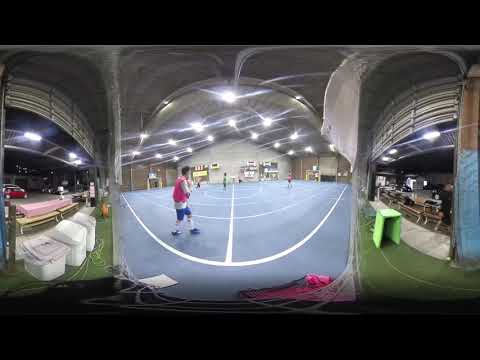This image appears to be a 360-degree photo or a fisheye lens capture, with black bars across the top and bottom and distortion warping the view. At the center of the shot, an indoor sports court, possibly a pickleball or modified tennis court, dominates the scene. The court itself has a light blue, somewhat clay-like surface, marked with white lines. A player, distinguished by a reddish-pink vest over a white shirt and dark blue shorts, is prominently positioned in the middle.

The surrounding environment features a large indoor structure illuminated by numerous ceiling lights, which due to the photo's distortion, emit bright glares and rays. On either side of the court, areas with lime green benches or stools and small tables are visible, one of which is adorned with a checkered white and red tablecloth. The left part of the image shows additional indoor sections that might resemble a parking garage, with various equipment and possibly a training table for injuries.